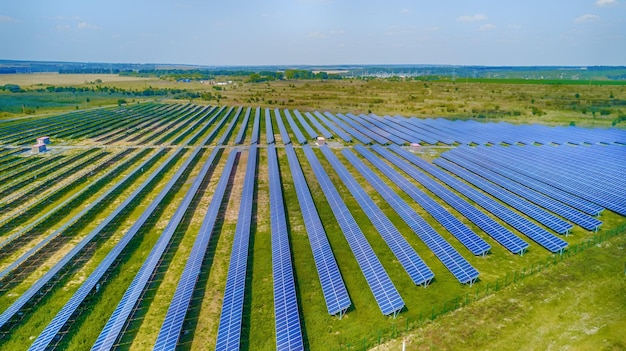This is an aerial angled view of an expansive solar panel farm consisting of two large fields filled with numerous rows of rectangular, blue solar panels outlined in white. The fields are divided by a small road that cuts through the area. Scattered across the fields are four small white structures, adding a sense of scale and functionality to the site. The fields are predominantly green with patches of brown where grass has withered, indicating some variations in the vegetation. In the bottom right corner, a large green fence can be seen lining the perimeter of the field. In the foreground, an empty field reminiscent of farmland stretches out, leading to the solar panels in the middle ground. The background features a landscape that could be either a distant body of water or hills and mountains, capped with a mostly clear blue sky adorned with a scattering of fluffy white clouds. Additionally, trees dot the surroundings, providing a natural contrast to the structured arrangement of the solar panels, and behind them, further back, buildings suggest a nearby inhabited area or town.